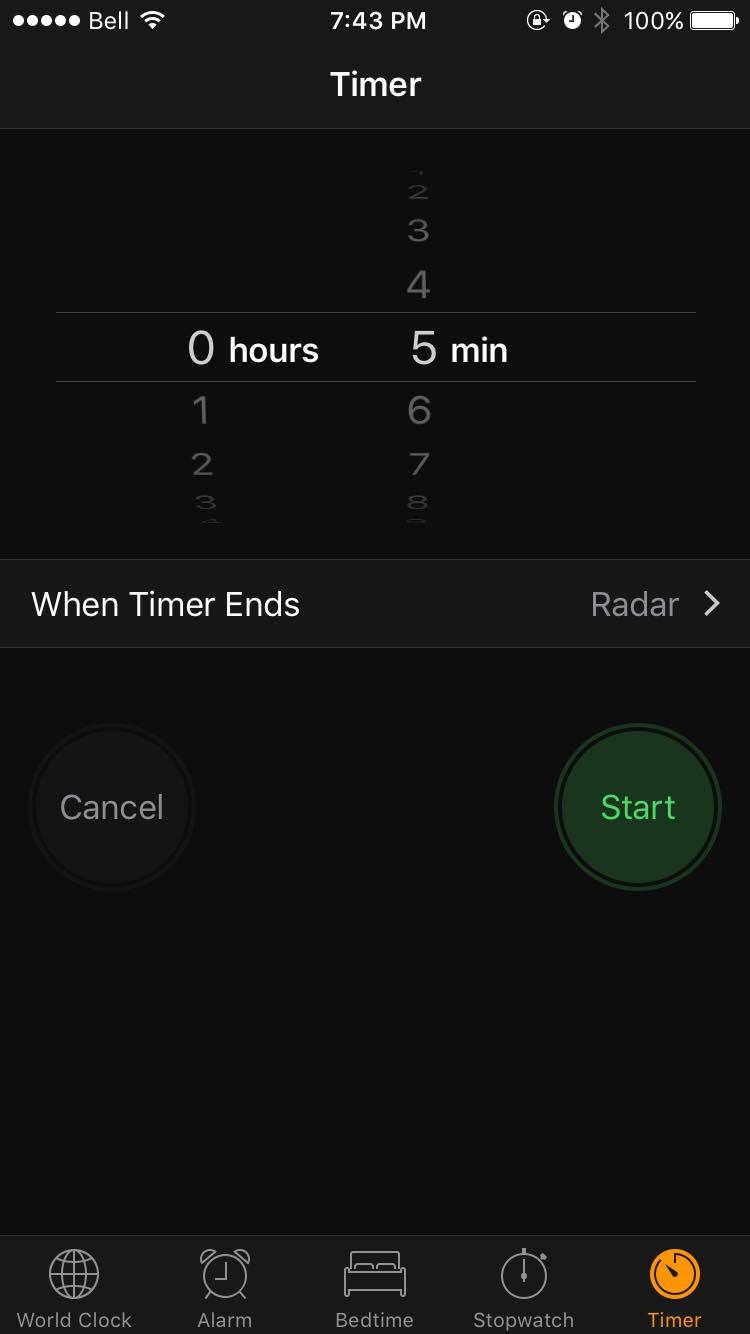A detailed and descriptive caption for the image would be:

"This image is a detailed screenshot of a smartphone displaying the Clock app. At the top of the screen, the word 'Bell' is prominently displayed, indicating the app's current mode. The volume is set to its maximum, as depicted by five filled dots located in the upper left-hand corner. The current time is 7:43 p.m., shown in the center of the screen. The phone's battery is fully charged at 100%, displayed on the top right.

The screen’s background is entirely black, providing a stark contrast to the white text and icons. The timer is set to zero hours and five minutes. Below this setting, there is a header reading 'When Timer Ends,' with the word 'Radar' next to it, which is a clickable option to the right.

At the lower part of the screen is a round black button labeled 'Cancel' on the left, and a round green button labeled 'Start' on the right. Beneath these buttons is a toolbar with clickable options including World Clock, Alarm, Bedtime, Stopwatch, and Timer. The 'Timer' option is highlighted in a goldish-yellow color, indicating that it is currently selected. Above the 'Bedtime' option is an image of a bed, and above the 'Alarm' option is an image of a clock."